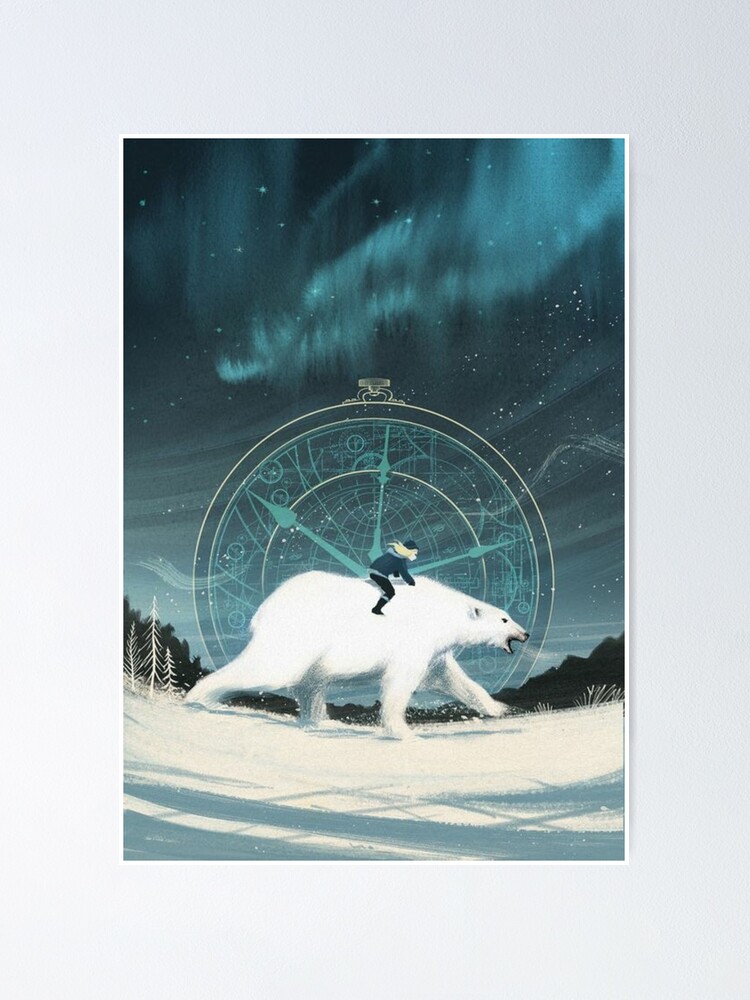The image is a vertically-oriented color illustration resembling a greeting card, framed by a light blue beveled matting with a white edge. The centerpiece is a color photo capturing a snowy, wintry scene with a large polar bear in the foreground carrying a rider, who could be a man or a boy, through a snowy landscape. The skies above them are a deep gray-blue, illuminated by vibrant, turquoise shapes reminiscent of the northern lights. Behind the polar bear, a subtle watermark of a stopwatch or compass with the winding part visible adds an intriguing element to the background. The landscape further showcases snow-covered trees transitioning to darker, unsnowed trees in the distance, while tiny white stars dot the sky, enhancing the ethereal atmosphere. The illustration invokes a sense of adventure and mystery, drawing the viewer in with its intricate details and captivating composition.